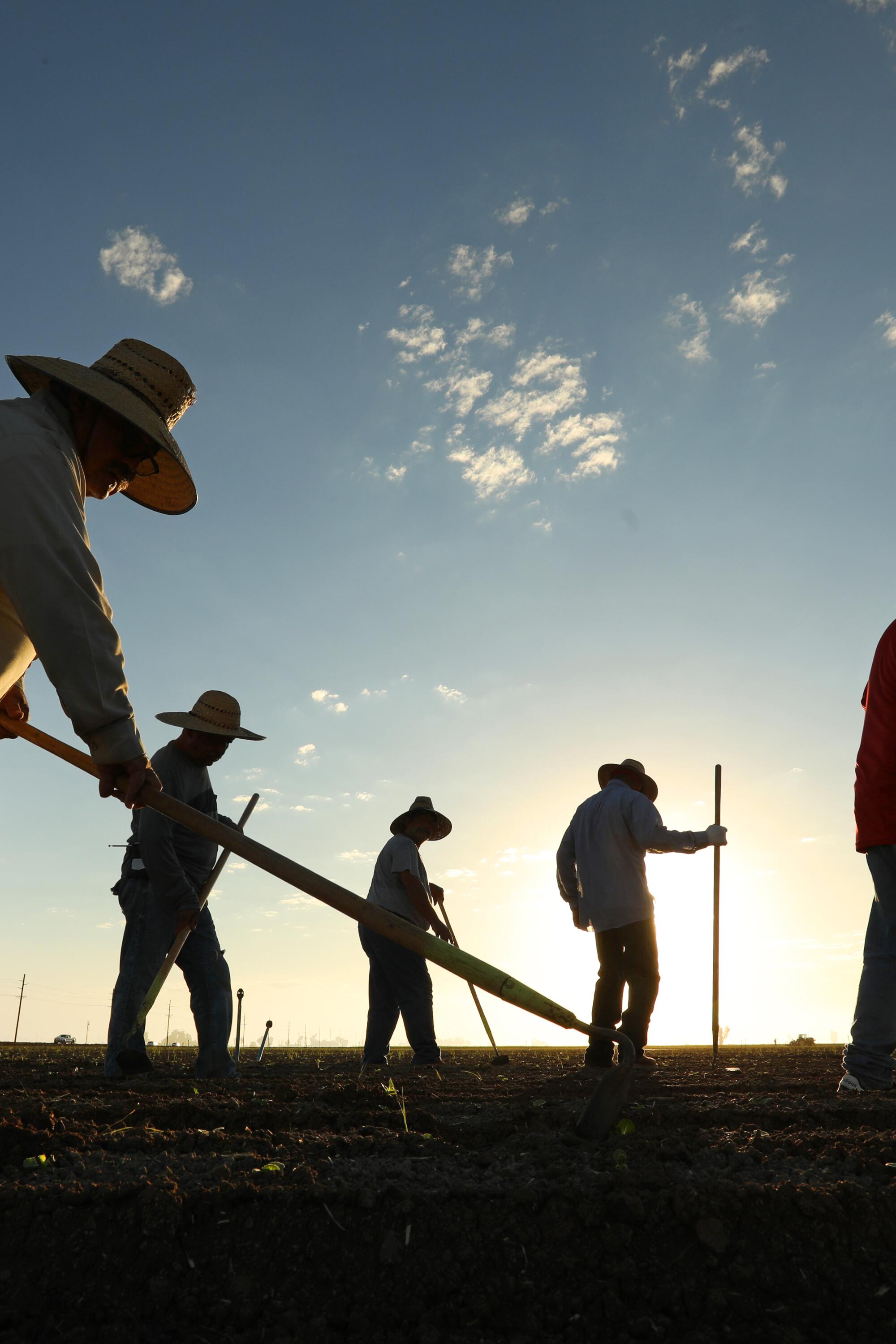The photo captures a vast, mostly blue sky with scattered, small clouds, creating a serene backdrop. Five farmers, most of whom appear to be men with one possible woman, are silhouetted against the backdrop due to the low angle of the sun, which is either rising or setting, casting a golden hue over the scene. These farmers, wearing straw hats and dressed in white shirts with jeans or khaki pants, are spread out across a flat, well-maintained field. The foreground features one farmer prominently using a hoe to till the soil, while others either hold their tools by their sides or use them for support. Power lines and distant vehicles are barely visible at the horizon, suggesting a rural setting. The lighting and composition emphasize the hardworking silhouettes of the farmers against the expansive and subtly illuminated sky, giving a sense of early morning or late afternoon labor.